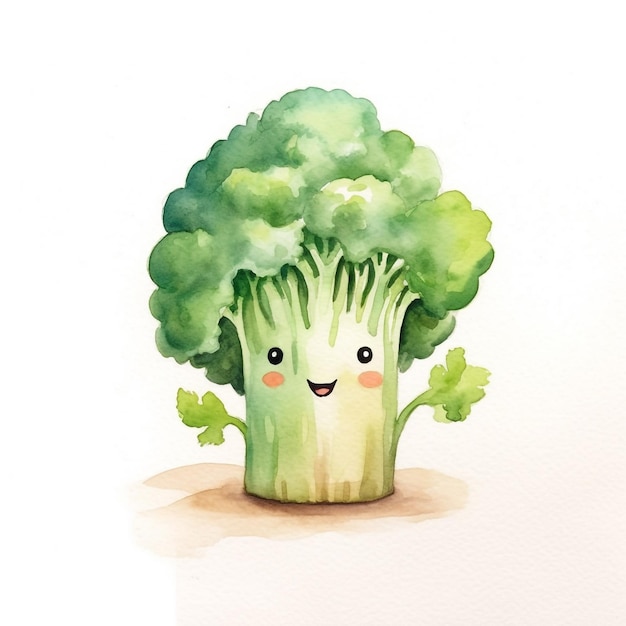This image is a whimsical, childlike illustration of a happy broccoli stalk that bears a strong resemblance to a small tree. The broccoli, presented in a watercolor or gouache style, stands tall with its bright green crown resembling a fluffy plume of hair. It has two lively arms made of smaller stalks extending outwards, each tipped with a small leaf, giving the impression of the broccoli waving joyfully.

The face of the broccoli is endearing, composed of two tiny black eyes and a wide, open-mouthed smile, epitomizing happiness. The cheeks display rosy red spots, adding a playful and friendly touch. Absent a nose, the simplicity of the facial features enhances its charm.

The broccoli is rooted in a patch of ochre brown ground, with the background transitioning from light pink to white, suggesting a soft glow possibly coming from the right side. The overall palette is dominated by greens and tans, contributing to a warm and inviting atmosphere, and aimed at encouraging children to view vegetables positively.

There is no text, artist signature, or notable illumination beyond the gentle gradient. This delightful illustration appears to be created with children in mind, promoting the idea of friendly vegetables.